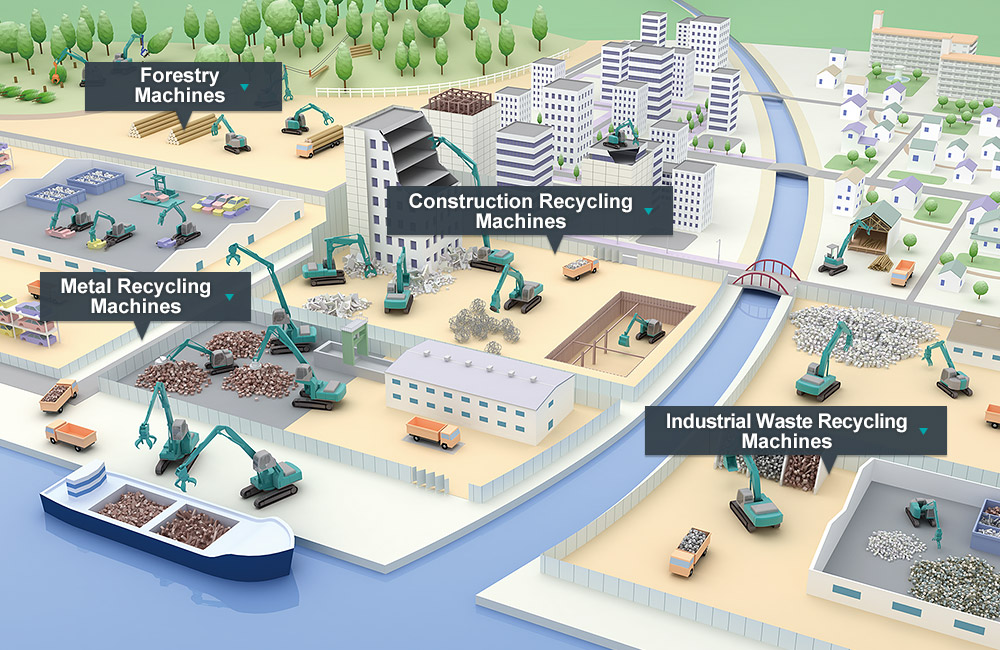The image depicts a pixelated aerial view of an industrial facility, resembling a scene from a city-building video game or a simplified diagram. This detailed illustration includes clearly labeled sections: a narrow blue canal runs through the center, curving off into the distance and connecting to a larger body of water. A notable feature is a large, flat boat docked in the shipyard at the shore. The land adjacent to the shore is paved and densely packed with various industrial buildings and machinery. Key areas are labeled with black text: on the top left, "Forestry Machines," indicating a segment potentially involving timber processing equipment; top center, "Metal Recycling Machines," suggesting an area dedicated to processing scrap metals; top right, "Construction Recycling Machines," highlighting an area for handling construction materials; and bottom right, "Industrial Waste Recycling Machines," detailing a section for processing industrial waste. The buildings are depicted in whitish-gray tones, giving a uniform, industrial look. Small bridges cross the canal, connecting different sections, and a small forest area is visible in the top left corner of the image, adding a touch of greenery to this otherwise industrial landscape.